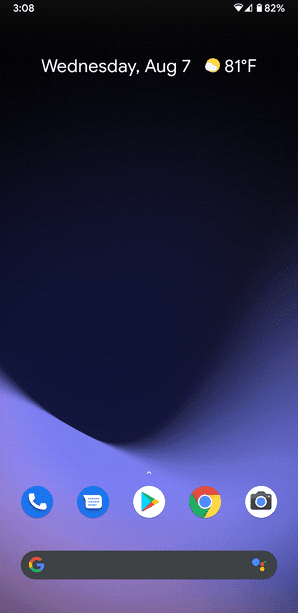Screenshot of a Smartphone Home Screen:

The screenshot captures the home screen of a smartphone. The phone appears to rise from the bottom left at an angle, climbs about 3 inches, dips slightly to the right by an inch, and continues upward off the right side, ending about 2 inches higher than where it started on the left.

The lower section of the screen is a light purple, transitioning to a darker hue toward the middle, before becoming entirely black near the top 2 inches. In the top left corner, the clock reads "3:08," displayed in white text. The top right corner shows the battery percentage at "82%" alongside the battery icon, a three-quarters-filled internet icon, and a similarly filled Wi-Fi icon.

Just beneath the time display, slightly right from the center, bold white text announces the date: "Wednesday, AUG 7." Beside this, a weather icon featuring a sun with a small overlapping cloud indicates a temperature of "81°F."

About 2 inches from the bottom, the screen includes a series of app icons: a blue circle with a white phone, a blue circle with a white text message icon, the Google Play app icon, the Google Chrome icon, and the camera icon. Directly beneath this line of apps is a gray search bar.

On the left side of the search bar is the Google "G," colored in red on top, yellow on the left, green on the bottom, and blue on the right. To the right end of the search bar, there's a series of smaller circles: a blue circle adjacent to a red circle, and beneath both, a smaller yellow circle.